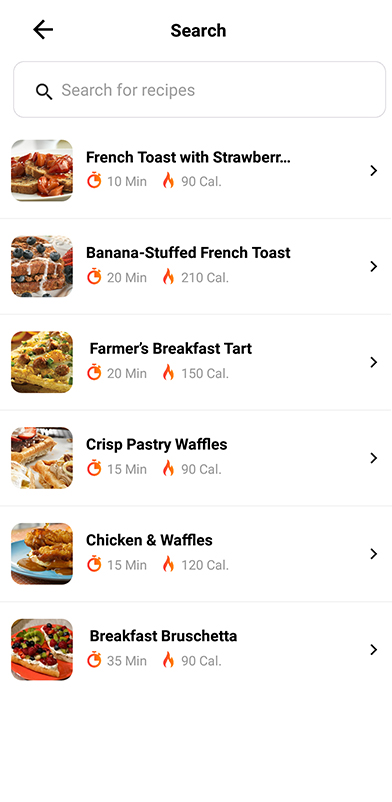In this image, we see a screenshot of a recipe app displaying a selection of breakfast recipes. The interface features a white background with a back button and a "Search" label at the top. Below this, there is a search bar prompting users to "search for recipes."

The list of recipes begins with "French Toast with Strawberries," accompanied by an image of the dish on the left. Next is "Banana Stuffed French Toast," with the corresponding image on the right. Following that is "Farmer's Breakfast Tart," featuring a picture of the food on the left. "Crisp Pastry Waffles" is shown below, with its image on the right. The list continues with "Chicken and Waffles," depicted with an image on the left, and finally, "Breakfast Bruschetta," also shown with an image on the left.

Each recipe entry includes preparation time and calorie information, providing users with an idea of the time investment and nutritional content of each dish.